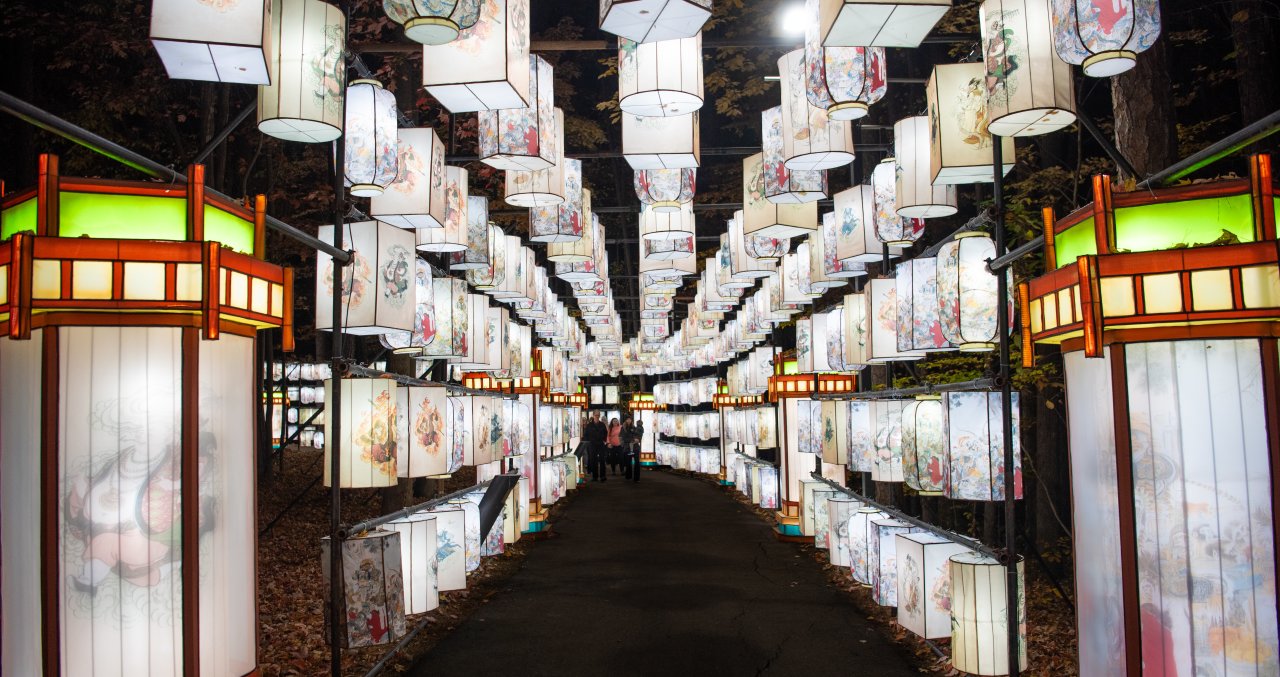This photograph captures a stunning exhibition of intricate lanterns displayed in a dark hallway. The composition features rows upon rows of beautifully designed lanterns, hanging both from the ceiling and lining either side of the walkway. The lanterns vary in shape, including squares, cylinders, and hexagons, and showcase an Asian-themed aesthetic with delicate designs—some depicting flowers, while others illustrate human figures. The lanterns predominantly have a light white or off-white hue, adding a serene glow to the scene. Prominent in the foreground are two larger lanterns, distinguished by a brownish-red wooden piece at the top, making them stand out from the rest. In the distance, a group of people, mostly dressed in dark clothing, are walking towards the viewer. Among them, a woman in a pink shirt stands out, adding a touch of color to the otherwise monochromatic scene. This image beautifully combines elements of art and light, creating an enchanting atmosphere.